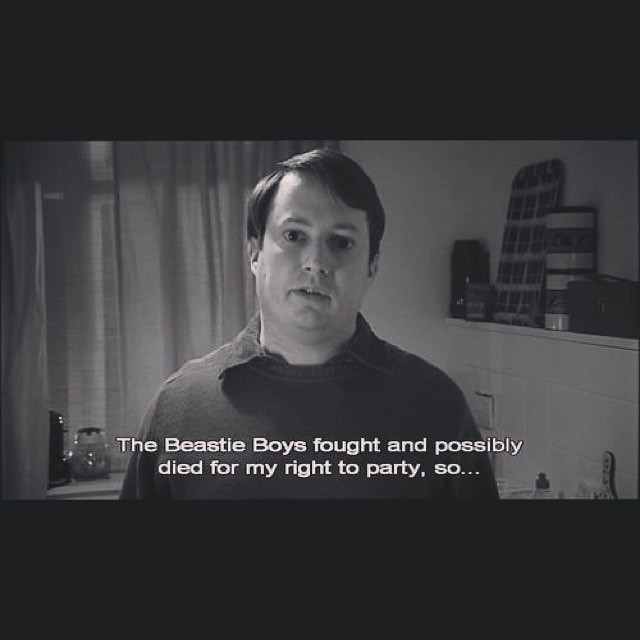This square black-and-white photograph, framed by black bands at the top and bottom like a film strip, captures a man staring directly at the camera with a serious expression. He wears a dark sweater layered over a collared shirt, his short, dark hair neatly parted. The setting appears to be a room with a window behind him, partially obscured by curtains. To his left, there's a shelf with various items, possibly toiletries or beauty products, hinting at a bathroom setting. Overlaid in white text near the bottom of the image, it humorously reads, "The Beastie Boys fought and possibly died for my right to par-tay, so..." The juxtaposition of the somber portrait and the lighthearted caption adds an element of wry humor, making it a likely candidate for social media or meme content.